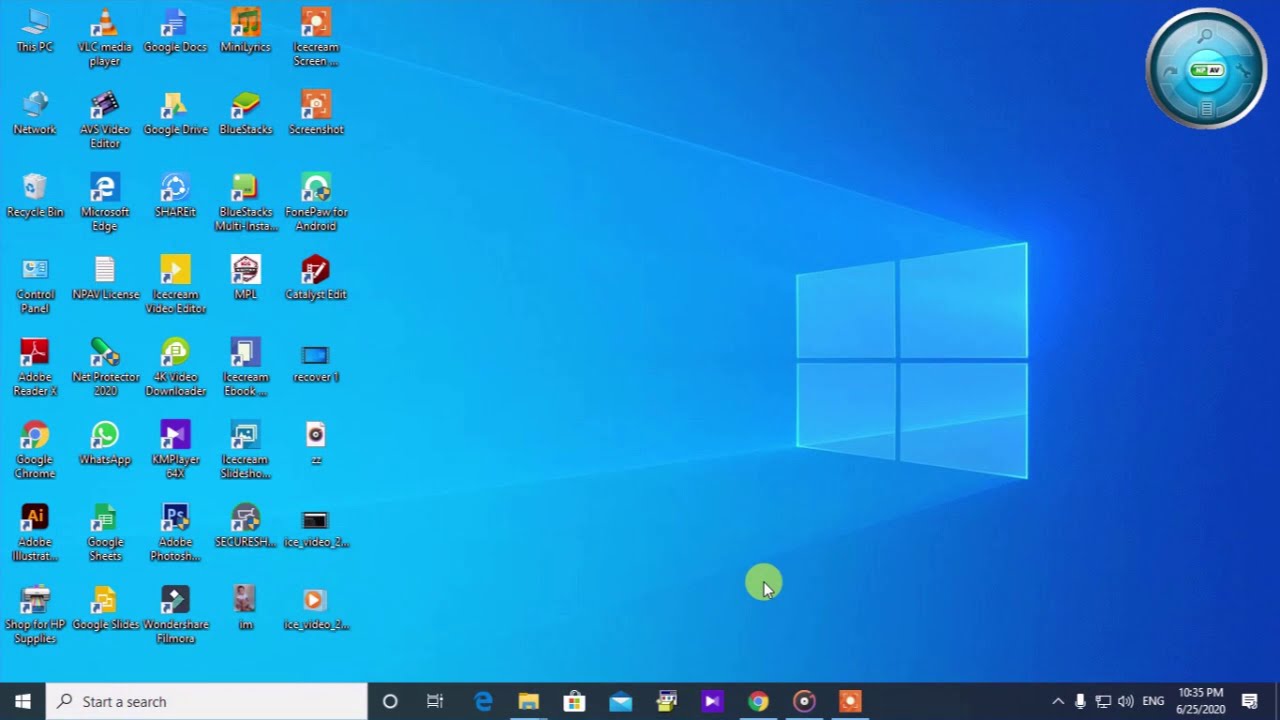This detailed screenshot depicts a typical Windows desktop as seen upon startup. The background is predominantly blue with a centered Windows logo composed of four squares with slight spaces between them. On the left-hand side, there are eight rows of icons, with five icons per row. The icons feature various colors and symbols, including familiar ones like Google Chrome in a circle with red, green, and yellow edges and a blue center. Other icons include a play button on an orange background, a recycle bin, and numerous other icons in shades of black, yellow, pink, and blue.

On the bottom left corner, a start search bar accompanied by a magnifying glass suggests that the user can initiate a search. Alongside, to the right of this bar, are several application icons like an E for Explorer, a folder, a shopping bag likely representing a Microsoft store, a blue envelope for email, and additional colored squares and circles representing various applications. Notably, a Windows Media Player icon is seen among them.

The lower right-hand corner of the screen displays the time and date - 10:35 PM, June 25, 2020, and confirms the language setting as English. The user's mouse cursor, highlighted by a green circle, is also visible on the screen. Overall, this image captures the essential elements of a freshly accessed Windows desktop, replete with assorted icons and standardized interface elements.